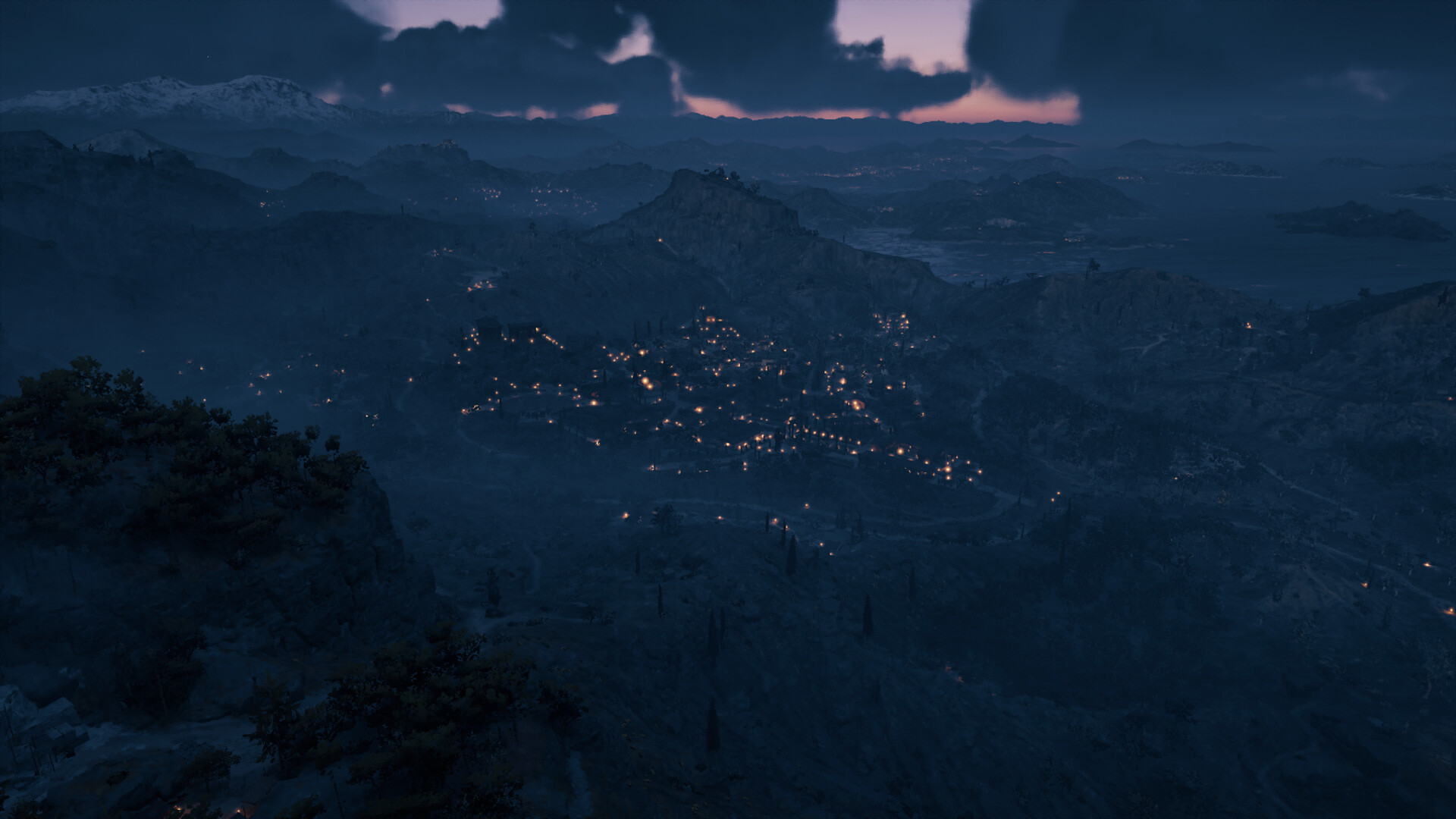In this atmospheric nighttime color photograph taken outdoors, the scene offers a captivating, albeit dimly lit, view of a city or town beneath a twilight sky. The upper portion of the image features a sky tinged with a pinkish-gray hue, interspersed with dark blue-gray clouds that stretch across the horizon. In the distance, a silhouetted range of mountains provides a majestic backdrop. Nestled at the foot of these mountains, a scatter of small orange lights punctuates the darkness, indicating the presence of buildings and homes in the town below. The foreground of the image, shrouded in near-impenetrable darkness, appears to contain some indistinct bushes, adding an element of depth and texture to the composition. Dominated by very dark blue tones, the photograph creates a somber yet mesmerizing nocturnal landscape, inviting viewers to peer into the hidden details within the shadows.